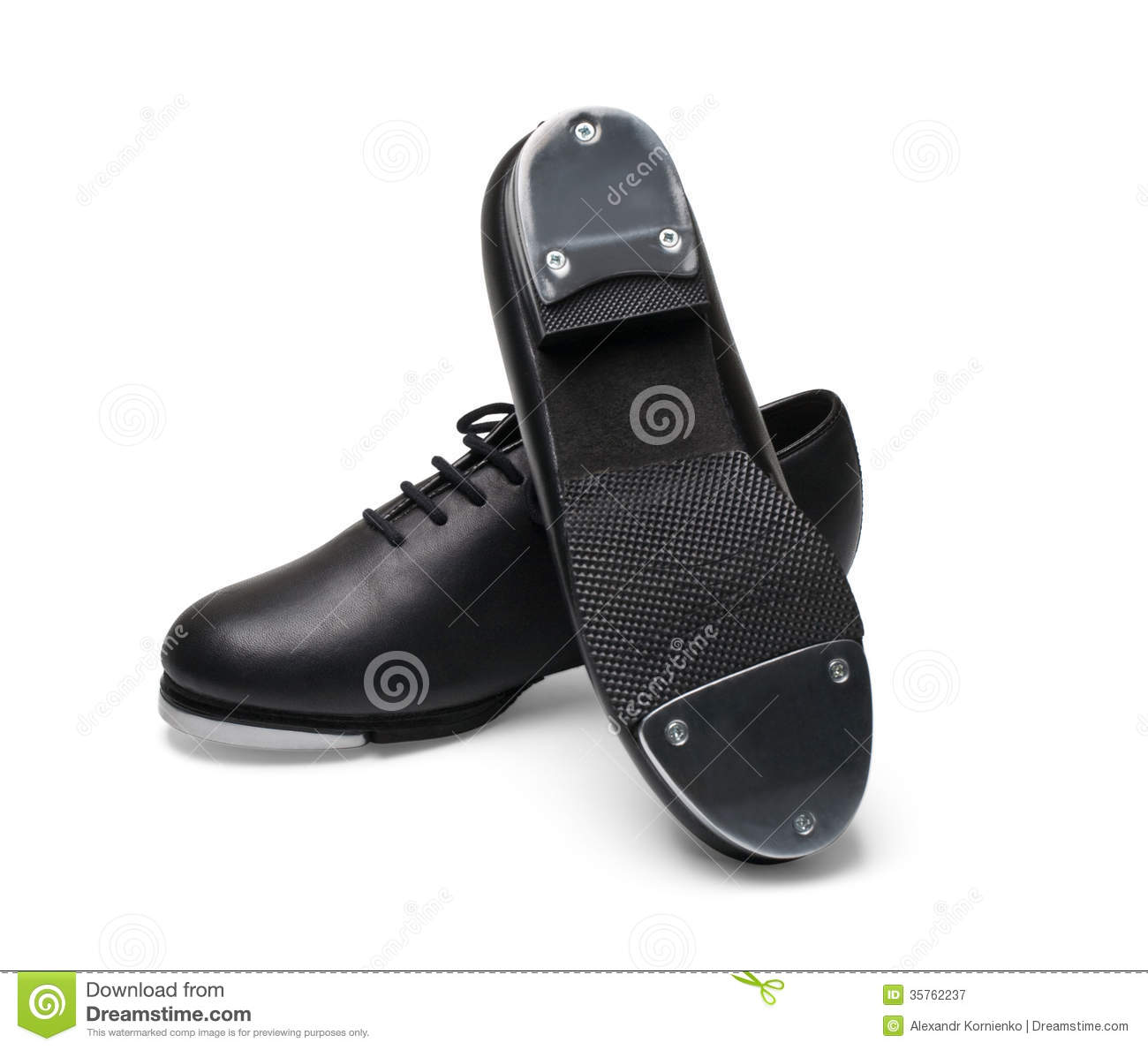This detailed stock image, image number 35752237 by Alexander Komienko from Dreamstime.com, features a pair of black lace-up tap shoes against a white background. One shoe is oriented upright, pointing towards the bottom left, while the other is turned upside down, revealing the intricacies of its sole. Both the heel and toe of the upside-down shoe are equipped with metal plates, each secured by three screws. The sole's uncovered areas have a textured grip, suggesting a rubber material. Overlaying the image is a watermark with checkered marks and the text "Dreamstime" along with a note stating "Download from Dreamstime: the watermarked comp image is for previewing purposes only," prominently displayed at the lower right corner.